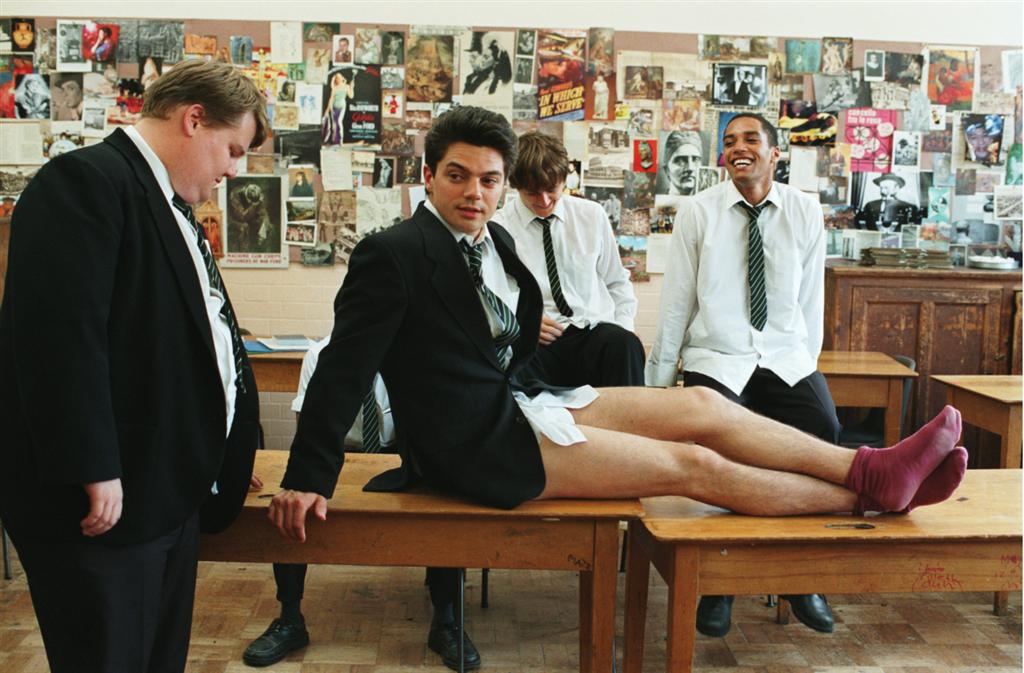In this intriguing and somewhat humorous image, a total of five men, all dressed in suits, are captured in what appears to be a college setting. Dominating the scene is a man sitting on top of two wooden desks pushed together, notably not wearing any pants, revealing his crimson socks. He sports a white button-down shirt, a tie, and a blazer. Next to him stands a larger man with dirty blonde hair, seen from his right side, clad in a white button-down shirt, a gray and black striped necktie, a black blazer, and black suit pants. Behind them, two other men are seated on a wooden desk, one being dirty blonde and the other African American, both dressed similarly in white button-down shirts, matching neckties, and black suit pants. A fifth man, partly visible, is seated further in the background. The atmosphere is light with one of the men sharing a good laugh. The background features a beige wall filled with what looks like pages from magazines, adding to the casual and whimsical setting. None of the men are looking directly at the camera, contributing to the candid, almost old-movie-like vibe.